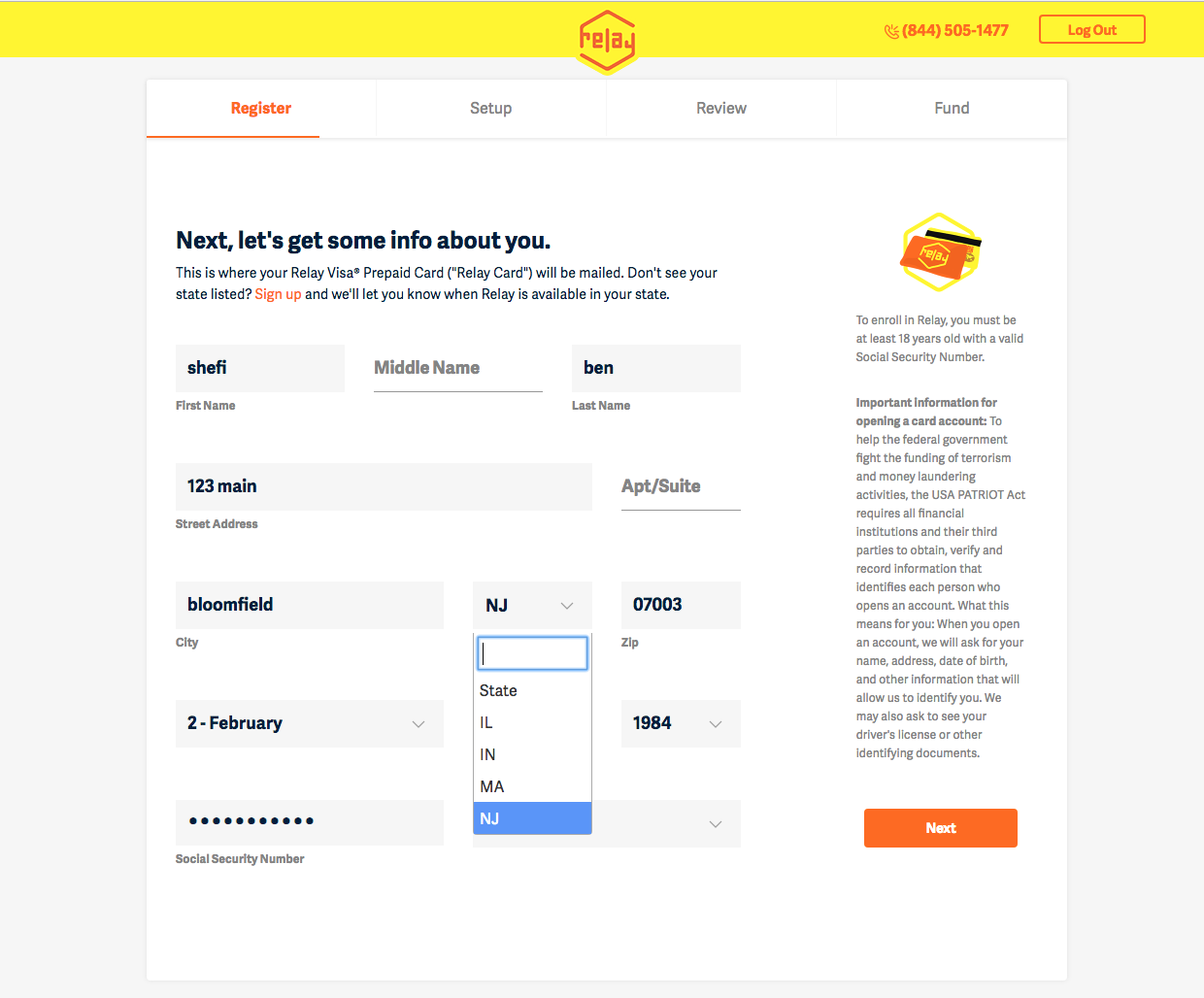The image depicts a registration page for the Relay website, characterized by a vivid yellow stripe across the top. At the center of this stripe, the Relay logo, rendered in red, stands prominently. On the right of this stripe, there is a small phone icon accompanied by the phone number 844-505-1477 and a logout button adjacent to it.

At the top of the page, four navigational categories are displayed: Register, Setup, Review, and Fund. The "Register" category is highlighted, indicating the active page. Below this, a section prompts the user with "Next, let's get some info about you," specifying that this is the address where the Relay Visa Prepaid Card (referred to as the Relay Card) will be mailed. It also addresses users who don't see their state listed, directing them to sign up to be notified when Relay is available in their state.

The page features several text boxes for user information, including fields for First Name, Middle Name, Last Name, Street Address, Apartment/Suite Number, City, State, Zip Code, Date of Birth, Year of Birth, and Social Security Number. The last field's label is obscured by a drop-down box from the State selection.

On the right-hand side, the Relay logo reappears along with instructions and important information about opening a card account. This section includes paragraphs outlining compliance with the US Patriot Act, concluding with an orange 'Next' button at the bottom, which directs users to the next step and provides explanations of terms and fees.